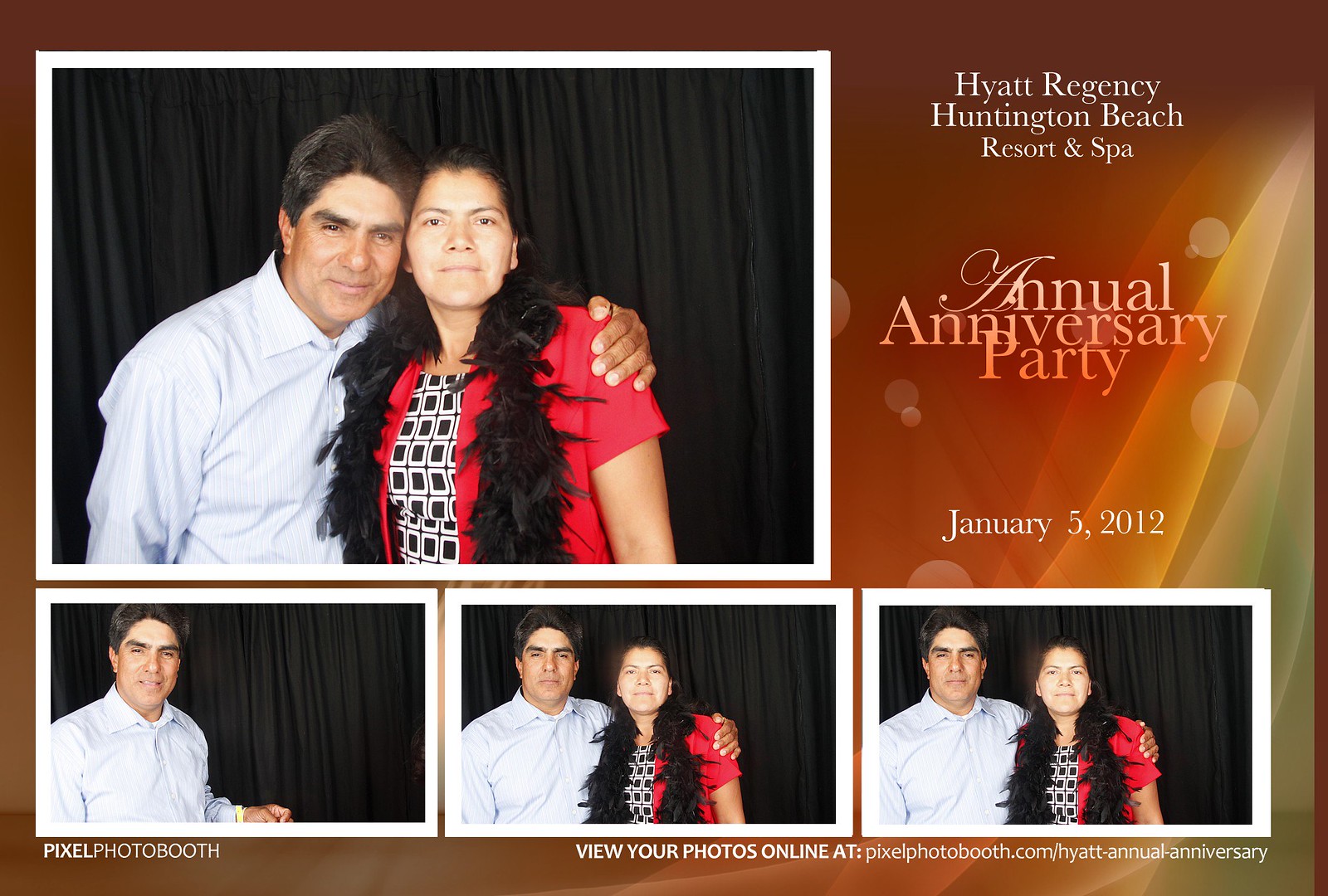This is a detailed description of a series of four photos taken in a photo booth at the Hyatt Regency Huntington Beach Resort and Spa Annual Anniversary Party on January 5, 2012. The photos capture a couple in their late 40s to 50s, posing against a black curtain backdrop. The man, with dark hair and likely Latino, is dressed in a light blue button-down shirt. The woman, also with dark hair, is dressed in a red short-sleeve cardigan over a black and white dress and accessorized with a black feather boa. The top left photo shows the couple together, smiling at the camera, while the remaining three photos at the bottom include a solo shot of the man on the left and two more pictures of the couple. The rightmost photos show them standing closely, the man with his arm around the woman, both sharing slight smiles or pleasant expressions. The event details and a message to view the photos online at pixelphotobooth.com are prominently displayed at the top and bottom of the image.